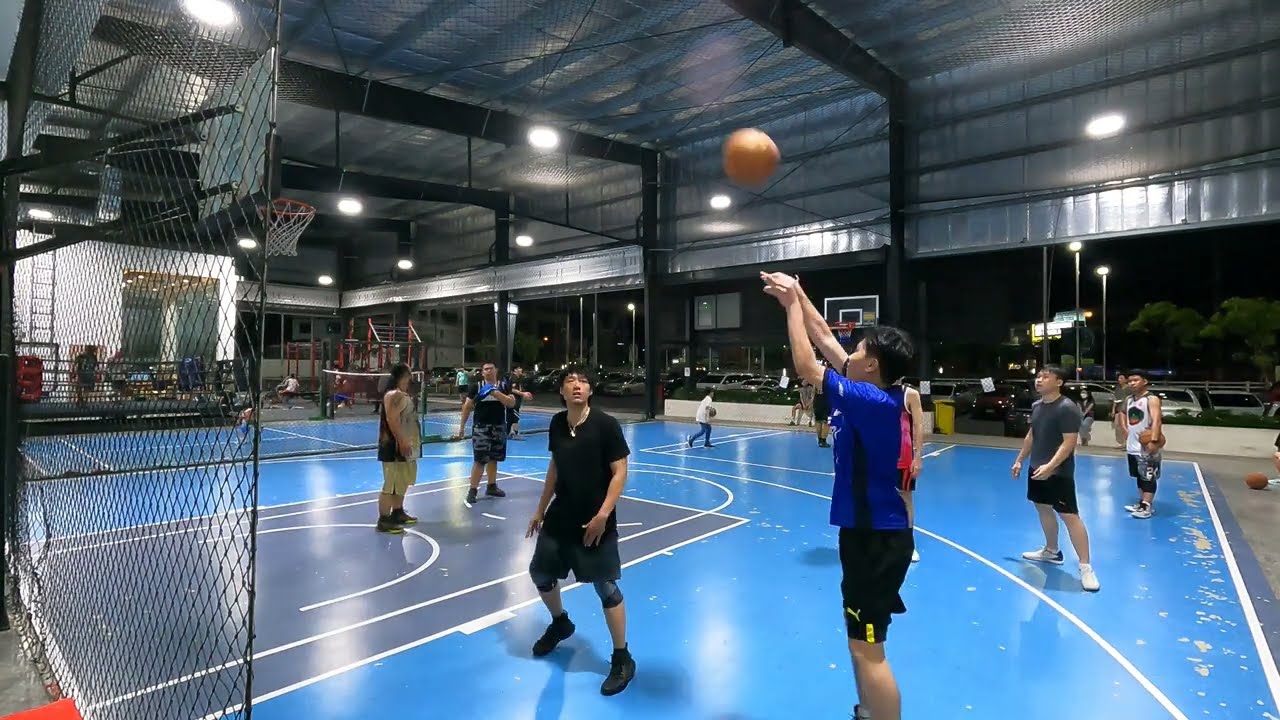The image features an indoor recreational area that combines elements of both indoor and outdoor spaces. The focal point is a bright blue basketball court located in the foreground, where several men are casually playing. The man closest to the camera is captured mid-shot, with his arms extended, wearing a blue shirt and black shorts. A man in a black shirt and blue shorts stands nearby, seemingly ready to rebound. The court's surroundings reinforce its casual use; the players are dressed in everyday sportswear rather than team jerseys, indicating an informal game. Beyond the court, large open areas and open doors reveal a parking lot with cars, dimly lit by streetlights, and the dark sky. The gym is equipped for various activities, as suggested by the nearby nets and the visible hockey layout on the floor. Lastly, the gym's far end showcases a long row of windows and additional equipment, highlighting the multi-functional nature of the facility.